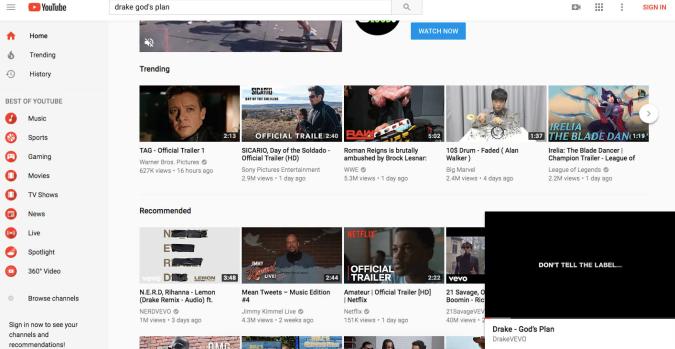This image captures a YouTube search results page for the query "Drake God's Plan," with "God's" incorrectly written with a lowercase "g." The following elements are visible in detail:

- **Top Navigation Bar**: Featured on the right side are three horizontal bars next to which is a red box with a white arrow and the text "YouTube."
- **Search Box**: Positioned centrally at the top with the entered search query "Drake God's Plan."
- **Right Icons**: A red sign and several other icons situated on the far right of the top navigation bar.
- **Left Sidebar**: Headers and categories include:
  - General Navigation: Home, Trending, History
  - Best of YouTube: Music, Sports, Gaming, Movies, TV Shows, News, Live, Spotlight, 360 Video, Browse Channels
  - Each category is accompanied by red icons, especially noted for Sports, Gaming, Movies, etc.
  
- **Main Content Area**:
  - Results primarily show thumbnail images from video trailers, music videos, and other multimedia content.
  - Specific Results: 
    - "Tag - Official Trailer #1 - Warner Brothers Pictures," uploaded 16 hours ago with view count details
    - "Sicario: Day of the Soldado - Official Trailer HD"
    - "Roman Reigns is brutally ambushed by Brock Lesnar"
    - "105 Drum-Faded Alan Walker"
    - "Irelia - The Blade Dancer - Champion Trailer (League of Legends)"
    - "N.E.R.D. (featuring Rihanna) - Lemon (Drake Remix)"
    - "Mean Tweets - Music Edition #4"
    - "Amateur - Official Trailer HD (Netflix)"
    - "Drake - God's Plan" in black with white letters stating "Don't tell the label" under the video.

Overall, the image showcases a comprehensive YouTube search results page, highlighting popular video trailers and music videos relevant to the search query.